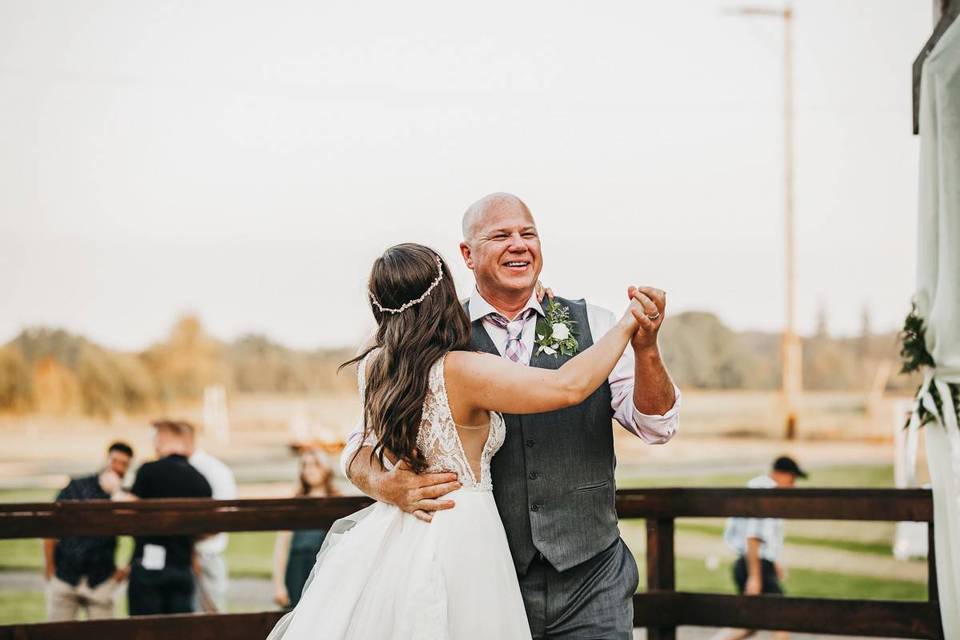In this detailed photograph, we observe a heartwarming father-daughter dance set against the backdrop of an outdoor wedding. The father, bald and smiling widely with eyes squinting, wears a gray vest over a pink shirt, complete with a pink and gray checkered tie and a green-stemmed, white-petaled flower on his chest. He graces the dance floor without a jacket, exuding a warm and approachable demeanor. His left hand clasps the raised hand of his daughter, while his right arm is lovingly wrapped around her waist. 

The bride, seen from the back, dons a white wedding dress accented with a delicate floral wreath crown in her grayish-brown hair. The dress features a beautiful floral pattern that adds an elegant touch to her radiant appearance. 

The background reveals a slightly blurred scene of reddish-brown autumn foliage, a gray sky, and indistinct rocky formations. Additional wedding guests mill about a short green grass lawn, with some appearing as a group of three engaged in conversation. Prominent among them is a blurry figure with a raincoat on the right side. Dark wooden beams of a fence frame the scene, and a tall lamppost protrudes in the distance, adding to the enchanting atmosphere of this special moment.